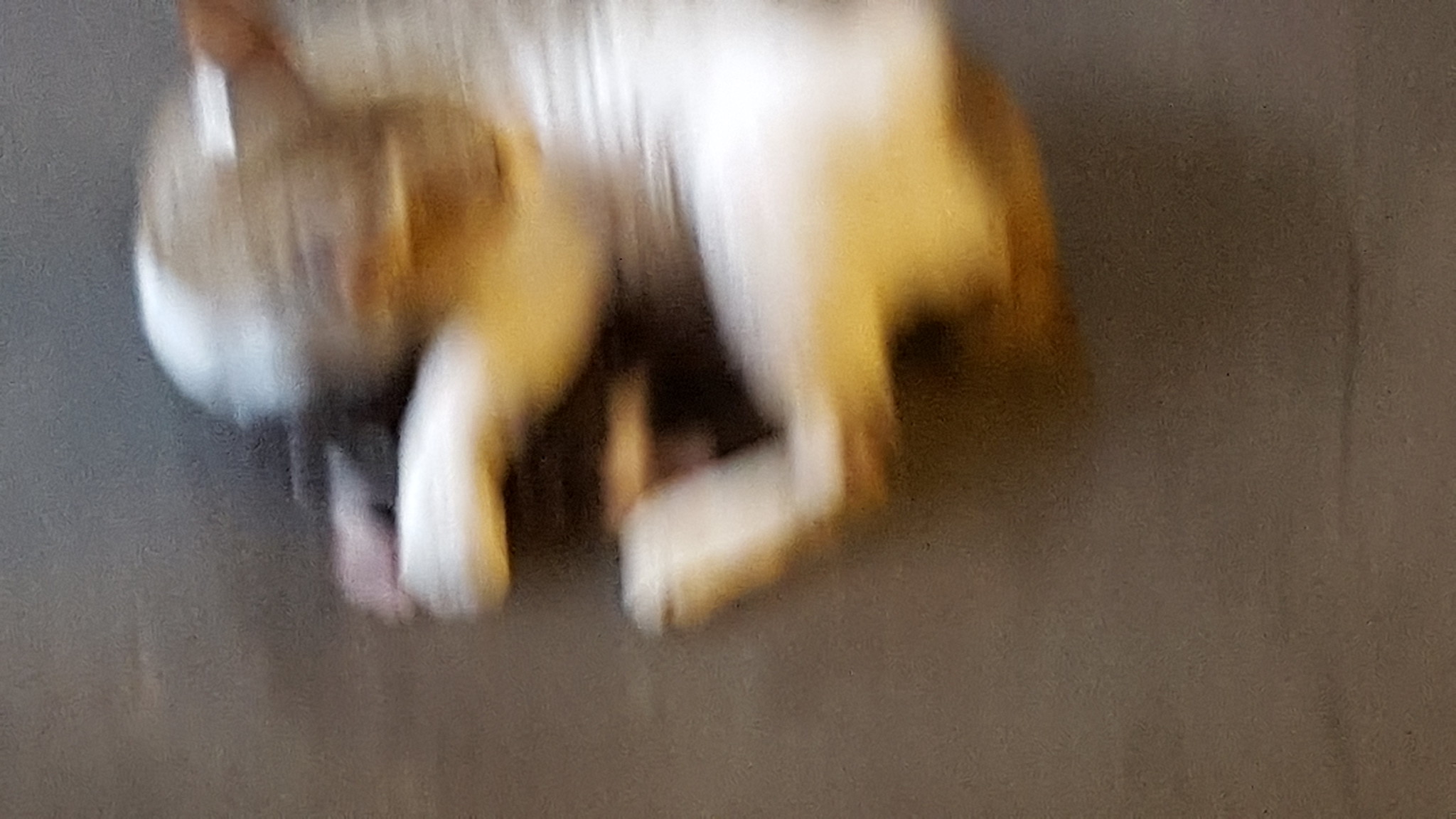In this blurry image, a small animal, most likely a kitten or possibly a hairless cat, is laying on its right side on a gray surface that could be industrial carpet or linoleum. The kitten, which is mainly white with distinctive brown markings, has its left side facing the camera. Its left ear and part of its face are brown, with a brown stripe running from its back to the top of its head. There is a brown tail visible and a brown patch near the elbow on its back leg. Curled up as if disturbed during rest, the kitten appears to have a dark brown or black toy between its legs, with a small white line at the bottom of the toy. Due to the poor image quality, details of the face and most of the body are unclear, but the general posture and colors can still be discerned.